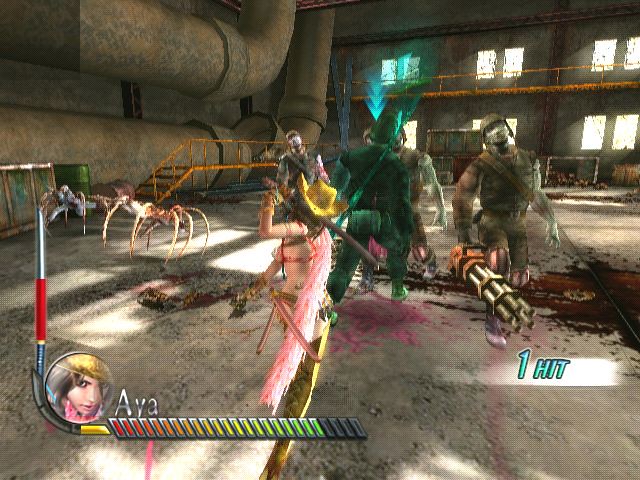The image is a screenshot from a video game set in an abandoned, industrial warehouse with a dark and foreboding atmosphere. The environment features large, brown and gray pipes on the left side near the top, and prominent windows and gray concrete-like walls. Yellow railings and catwalks crisscross the top right and left sides of the scene. The floor appears to be made of gray and brown concrete or stone. 

A central figure, a woman named Aya as indicated by the game interface, is displayed with a health bar in the bottom left corner, showing a gradient of red, yellow, orange, and green colors. Aya is depicted with a circular icon of a female face beside her name. She wears a yellow cowboy hat, a pink scarf or cape, a red bra, and yellow boots, and she is holding a sword. 

In the game scene, several hostile enemies are visible, consisting of large armored figures in brown, gray, and dark green, along with tarantula-like spiders that are brown and white. The screen also shows a combo counter or hit marker with the text "one hit" on the right side, highlighted in teal, indicating that Aya has just made an attack. The background features a mix of beiges, browns, and darker colors, with some elements like orange fencing adding to the eerie and desolate setting.